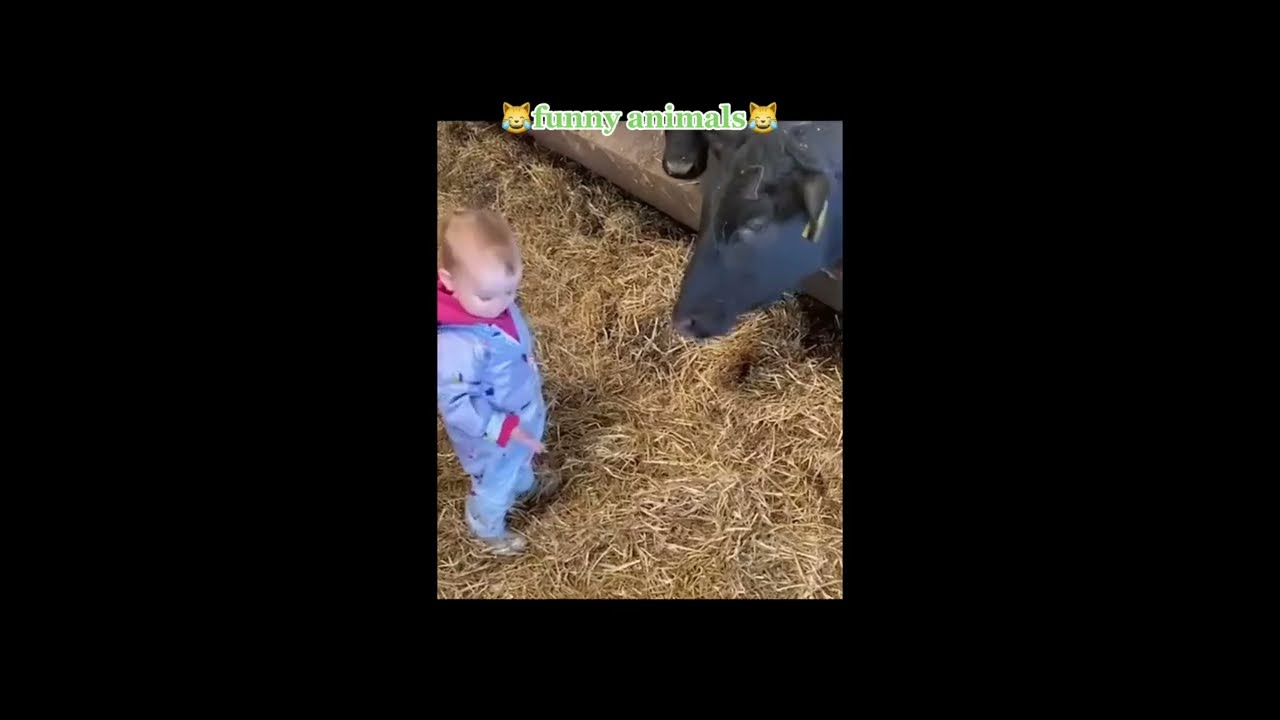The photograph depicts a scene bordered by a large black rectangle, creating a frame around the central content. Centered within this frame is a square image featuring a small child, presumably a toddler, dressed in a pink and purple outfit (with some confusion about it being blue) standing amidst a bed of hay. The toddler is looking down at their hand, while on the right side of the image, a curious black cow's head extends from a gated area or behind a barrier, peering towards the child.

Above this image, in green letters, are the words "Funny Animals", flanked by two images of animals laughing with tears, likely cats. The humorous and playful theme suggests a focus on the child and animal interaction set against a stark contrasting black border and background that underscores the vibrant scene within. There's a cement floor visible below the cow, adding to the rustic and farm-like setting.